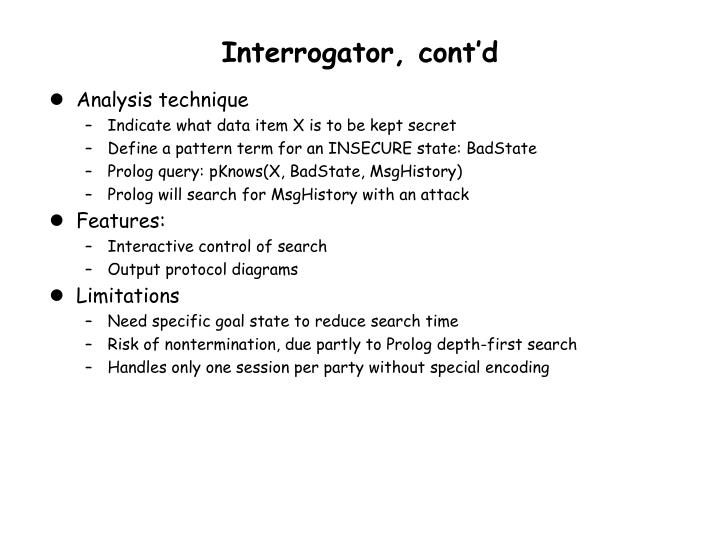The image is a text slide with an all-white background and black text. At the top-center in bold black letters, the heading reads "Interrogator, C-O-N-T'd," indicating it is a continuation. The content is organized into three main bullet points (analysis technique, features, and limitations), each followed by several indented sub-points marked with dashes.

The first main bullet point, "Analysis Technique," includes:
- Indicate what data item X is to be kept secret.
- Define a pattern term for an insecure state: bad state.
- Prologue query: P knows (X, bad state, MSG history).
- Prologue will search for MSG history with an attack.

The second main bullet point, "Features," includes:
- Interactive control of search.
- Output protocol diagrams.

The third main bullet point, "Limitations," includes:
- Need a specific goal state to reduce search time.
- Risk of non-termination, partly due to Prologue's depth-first search.
- Handles only one session per party without special encoding.

Circular bullets precede the main points, and dashes precede the sub-points. The text is aligned down the left side of the slide, creating a clear and structured layout.